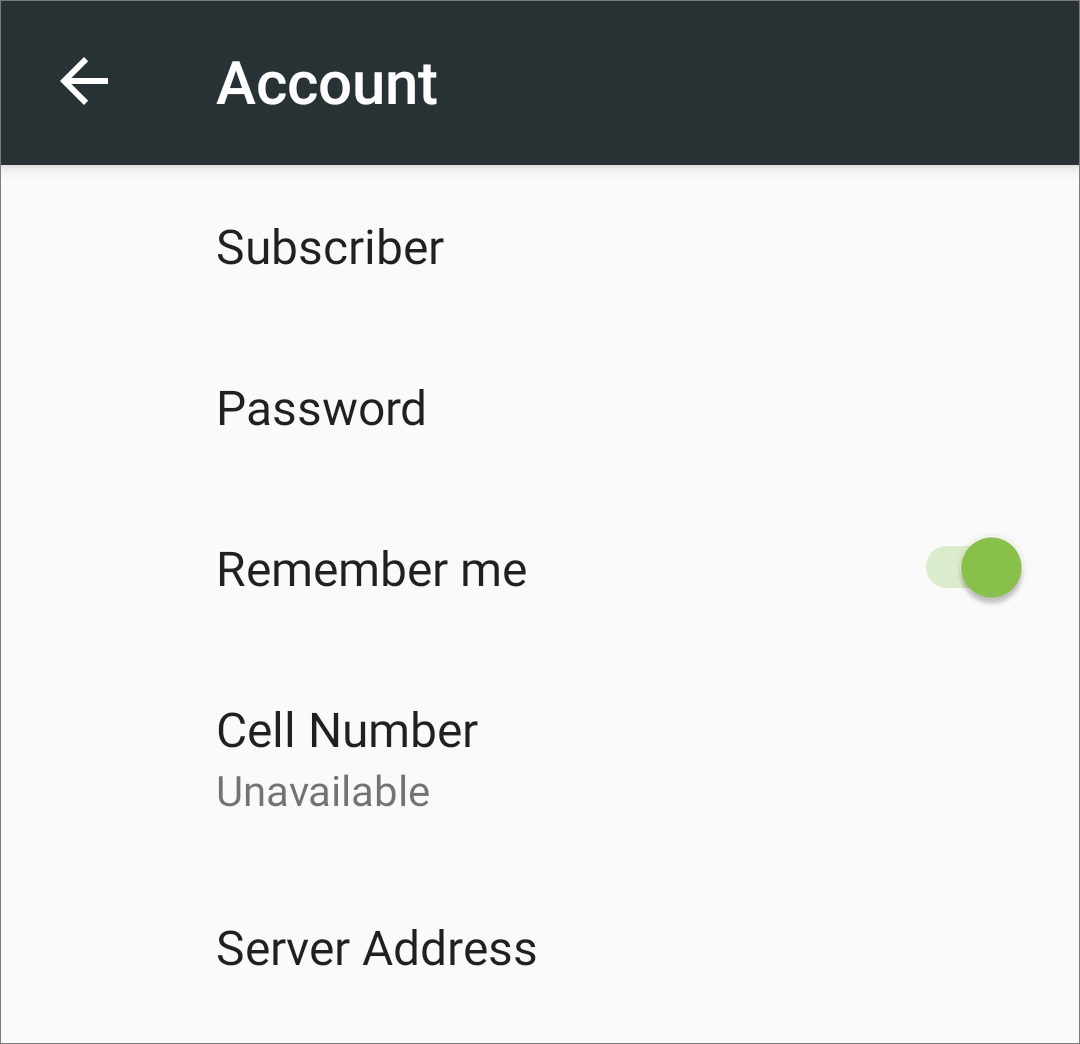The image appears to be a screenshot taken from a smartphone, showing the interface of an app's account settings page. The top 10% of the screen features a dark gray, almost black, bar with the word "Account" prominently displayed in large white text. To the left of the word "Account," there's a left-pointing arrow, also in white, likely a navigation icon to return to the previous screen.

Below this bar, the background changes to white and contains a series of five categories arranged vertically on the left side of the screen. These categories, listed from top to bottom, are labeled in black text as follows: "Subscriber," "Password," "Remember Me," "Cell Number," and "Server Address."

To the right of the "Remember Me" label, there is a green toggle switch, indicating the option to enable or disable the feature. Directly below the "Cell Number" label, the word "Unavailable" is displayed in a lighter, dark gray color, signifying that no cell number is currently associated with the account. Finally, the "Server Address" category is positioned at the bottom of this list, completing the account settings overview.